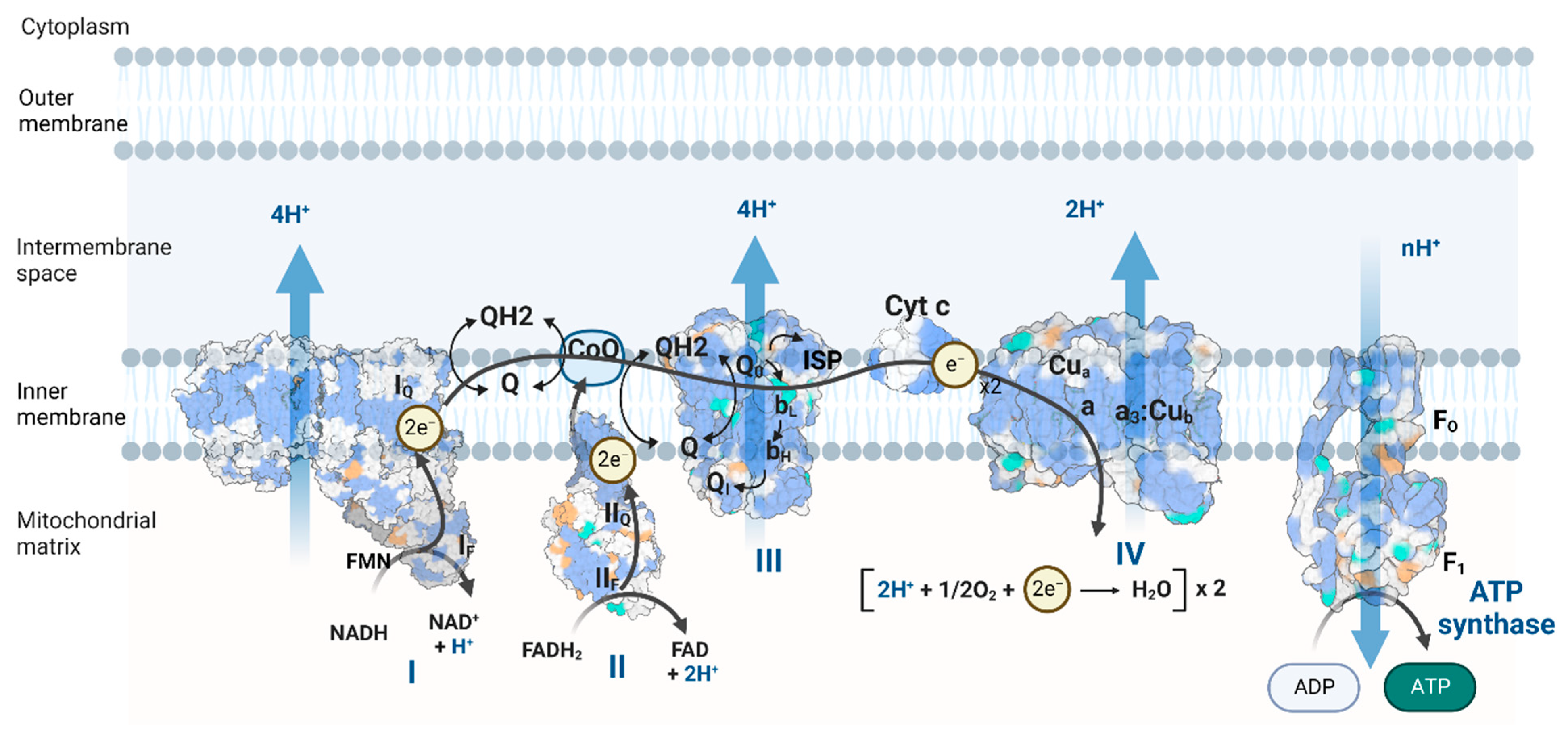This infographic depicts a detailed scientific chart focused on biological processes within cellular structures. On the left side, it lists labels from top to bottom: cytoplasm, outer membrane, intermembrane space, inner membrane, and mitochondrial matrix. The bottom of the chart is lined with various mathematical equations and formulas such as NADH, NAD+, FADH2, and FAD+2H. 

The central portion of the chart features several blob-like shapes adorned with blue, white, and orange dots, each representing different molecular entities or interactions. Blue arrows within these blobs predominantly point upward, symbolizing a particular direction of action or process, except for one blob on the far right where the arrow points downward. One of the blobs parallel to the listed labels on the left side lacks an upward arrow. Scattered across and within these blobs are additional equations, including FMN and electron transport components. On the lower right-hand side, two pill-shaped icons labeled ADP and ATP are situated just below the term "ATP synthase," indicating their roles in the cellular energy production pathway. This chart appears to illustrate complex biochemical pathways and molecular interactions involved in cellular respiration.